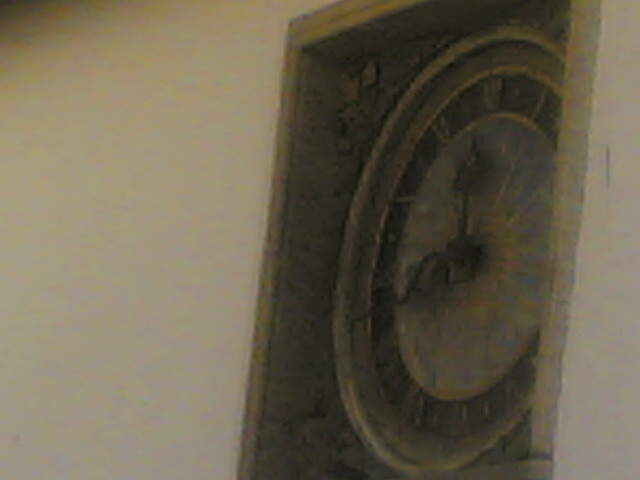A highly blurry and partially obscured image showcases a portion of a clock against a grayish lilac background. The upper left corner of the background exhibits a slight brown tint. Central to the composition is an upright rectangle bordered in light tan. Within this rectangle lies a darker gray area, which further encloses a beveled circle in a mid-gray tone. 

Inside the beveled circle, a darker, inner circle marks the beginning of the clock face. This inner circle contains a ring displaying Roman numerals; however, due to the image's blurriness, not all numerals are distinguishable. The 12 and 1 at the top are visible, as well as possibly the 5 and 6, but numbers on the right-hand side are much less discernible.

The central part of the clock face, where the hour and minute hands are located, is a lighter gray. The clock’s elaborate and scrolling hour and minute hands, rendered in dark gray, are distinctly visible, yet there is no second hand present in the image.